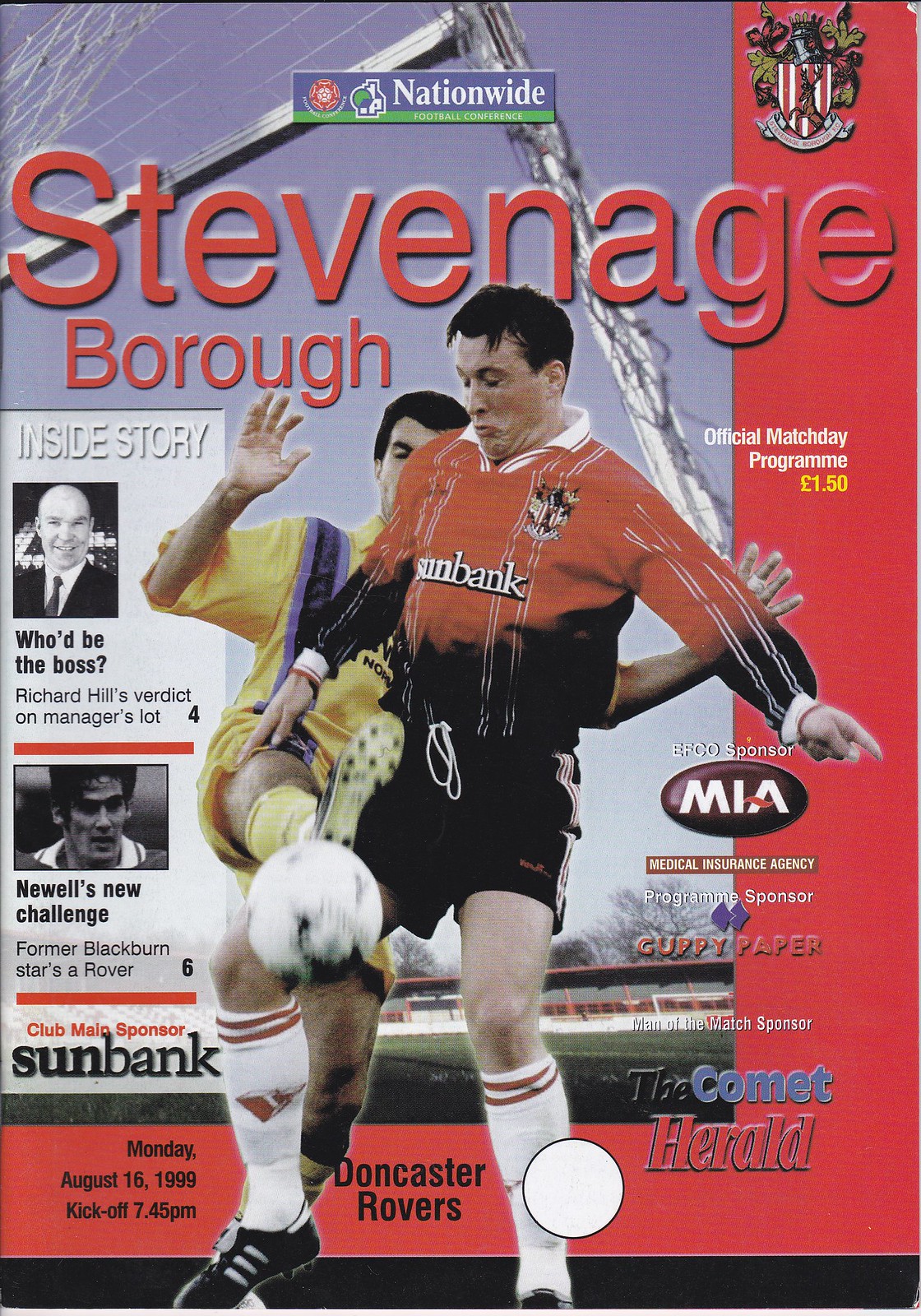The magazine cover features a central photo of two soccer players in action. One player, wearing a yellow jersey, is in the process of kicking the ball, while the other, donning a Sun Bank jersey, attempts to intercept. Above them, the title "Stevenage Borough" is prominently displayed in red text, along with a small box indicating "Nationwide Football Conference." The upper right corner showcases a football club crest, while the left side features various text snippets and photos, including an inset about Richard Hill's verdict on the manager, and details of Newell's new challenge, highlighting former Blackburn Stars Rover 6. The bottom right corner notes the "Comet Herald," along with the date and time of the fixture: Monday, August 16, 1999, kickoff at 7.45pm against Doncaster Rovers. Additional sponsor logos and names such as NIA (Medical Insurance Agency) and Guffey Paper are seen on the right margin. The cover has an aged, worn appearance, with an L-shaped red border on the left side.